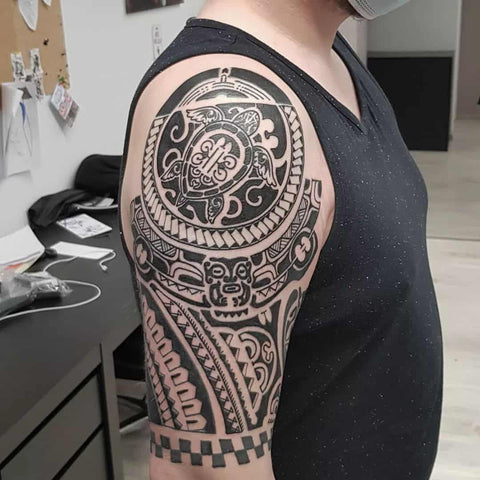This photo captures a detailed view of a person from the neck down to about the waist area, focusing especially on their right shoulder and upper arm. The individual is slightly right of center in the photo, facing rightward and wearing a gray, V-neck shirt. The image also shows a hint of a white face mask above the neck, while the person's head is mostly out of frame, revealing only a small part of their chin. The black tattoo on the right shoulder is strikingly intricate, featuring a prominent circular emblem with possible symbolic content, surrounded by geometric shapes and a possible depiction of a turtle, evoking Samoan or Hawaiian tribal designs. Beneath the circle is a half circle that loops from the bottom left to right, followed by more geometric motifs. Notably, the design concludes just above the elbow with a black and white checkered pattern. The background reveals a white wall adorned with a bulletin board extending out of view at the top left, and a black desk laden with various items, including a USB charger, contributing to the room's clean and orderly appearance.